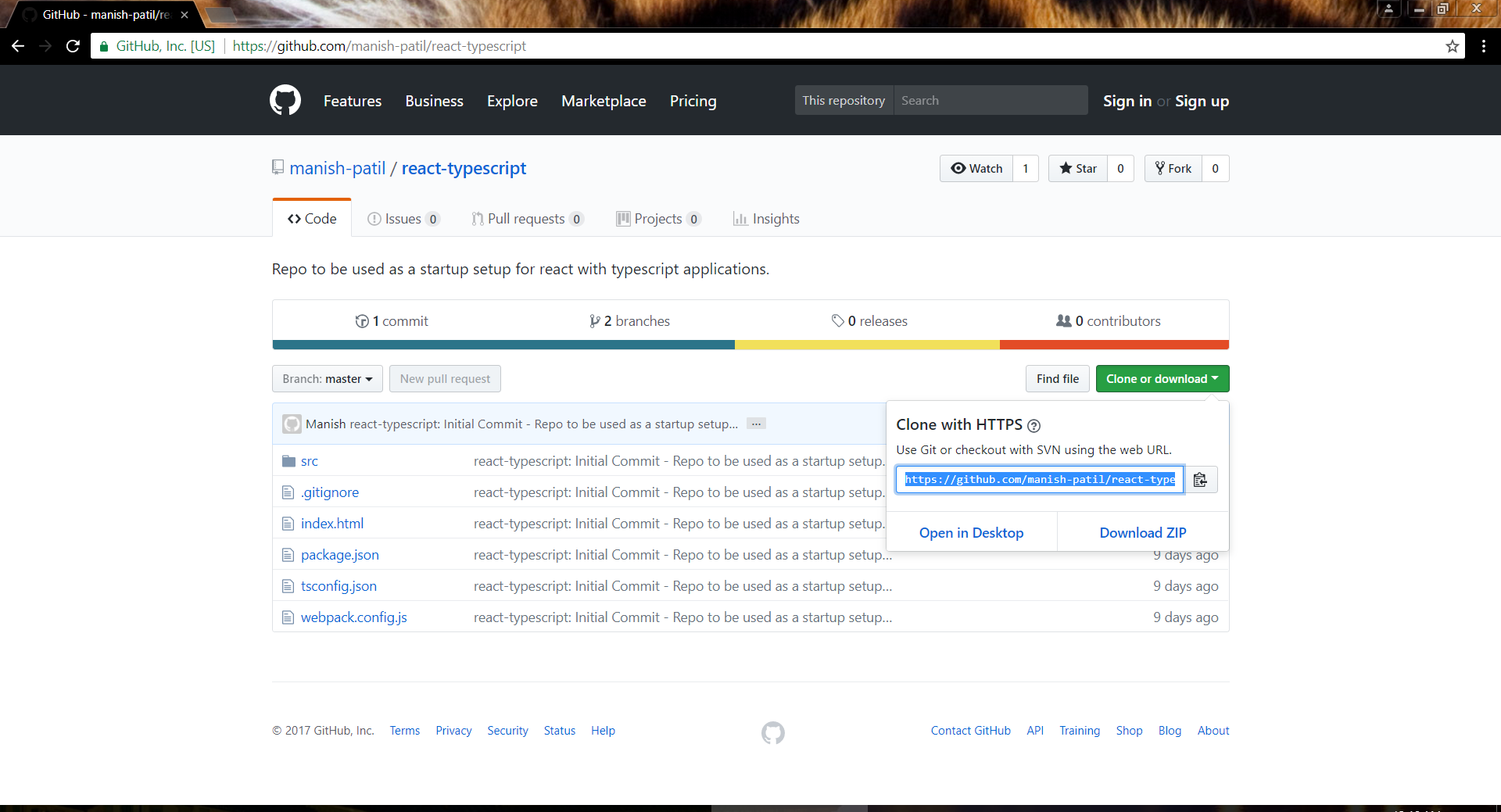In the image, the open webpage is GitHub, accessible via the URL github.com. The main page has a sleek black background header with white text. On the top left of the header, there are navigational links that read: Features, Businesses, Explore, Marketplace, and Pricing. An iconic cat logo also resides on the top left. On the top right, there's a search box and the options to sign in or sign up.

Below this header, the left section highlights "Manish Patil" and "Reactive TypeScript" written in blue. The top right section beneath the header shows the repository statistics: watch (1), star (0), and fork (0). Beneath "Manish Patil," there are various tabs: Code, Issues, Pull Request, Project, and Insights, with the "Code" tab currently highlighted.

The repository description states, "Repo to be used as a startup setup for React with TypeScript applications," accompanied by details: 1 commit, 2 branches, 0 releases, and 0 contributors. A colored line sits below these details, displaying dark green, yellow, and red segments. At the bottom section, it indicates branch: master, and includes an option for a new pull request.

There is a table listing different files and directories in the repository: SRC, .gitignore, index.html, package.json, tsconfig.json, and webpack.config.js – all written in blue. On the right side, there's a "find file" button in gray, and a "clone or download" button, which is green and white. Upon clicking "clone or download," a dropdown appears, displaying "Clone with HTTPS" and a note: "Use Git or checkout with SVN using the web URL." The URL provided is github.com-partil-react-typescript. Two options below the dropdown, written in blue, are: "Open in Desktop" and "Download ZIP file."